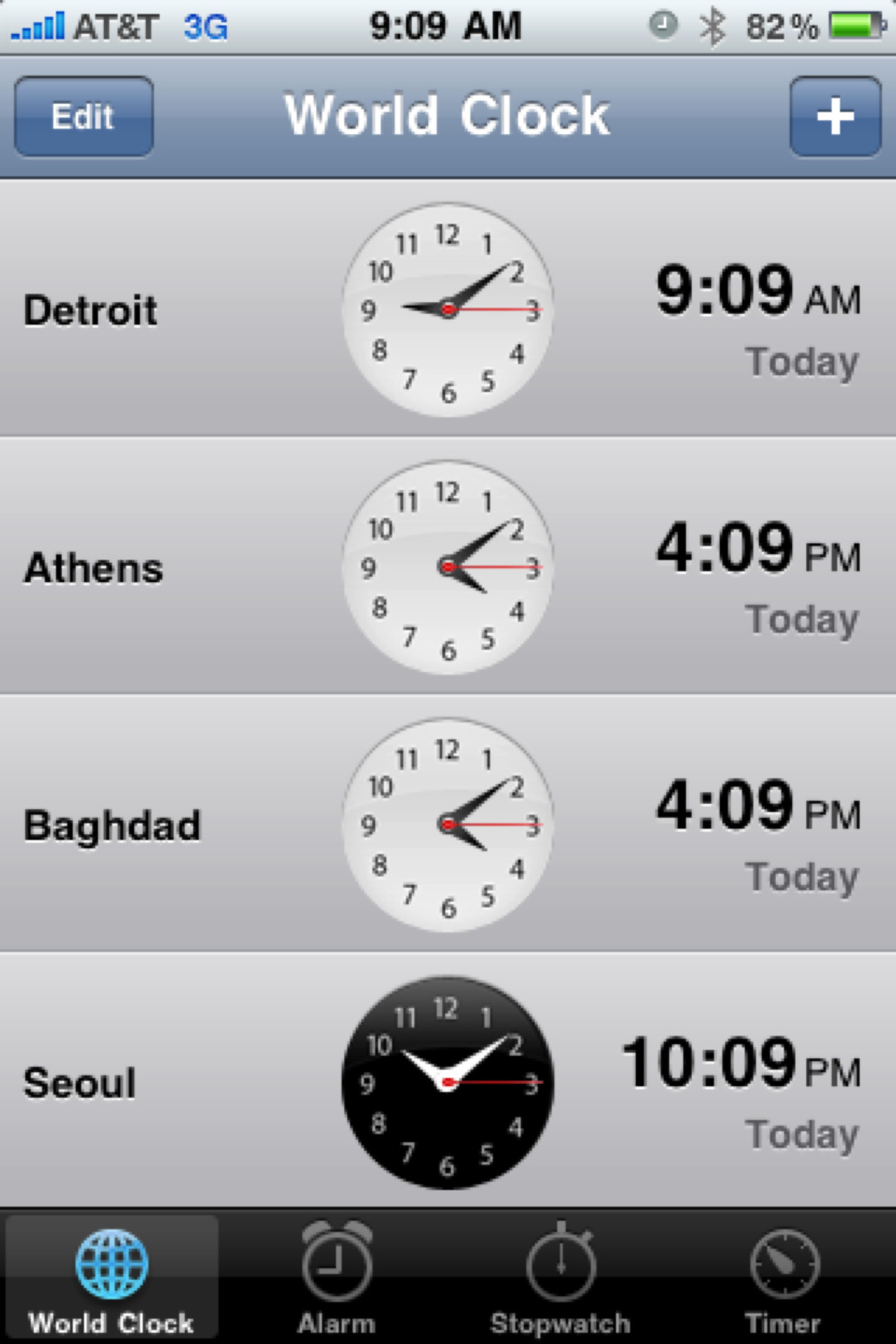The image is a screenshot taken from an older iPhone, displaying the World Clock app at 9:09 a.m. The top bar shows typical smartphone indicators: "AT&T 3G," an alarm icon, Bluetooth, and a battery level at 82%. The World Clock interface is highlighted in a blue box with white text, reading "World Clock" in the center, a plus sign (+) on the right, and "Edit" on the left. Four times are listed in black font: Detroit at 9:09 a.m., Athens at 4:09 p.m., Baghdad also at 4:09 p.m., and Seoul at 10:09 p.m. Each city's time is represented by a corresponding clock face, where the Seoul clock is distinctively black with white hands, possibly indicating nighttime. At the bottom of the screen, four navigational tabs are visible: World Clock (illuminated in blue to show it's the active tab), Alarm, Stopwatch, and Timer.